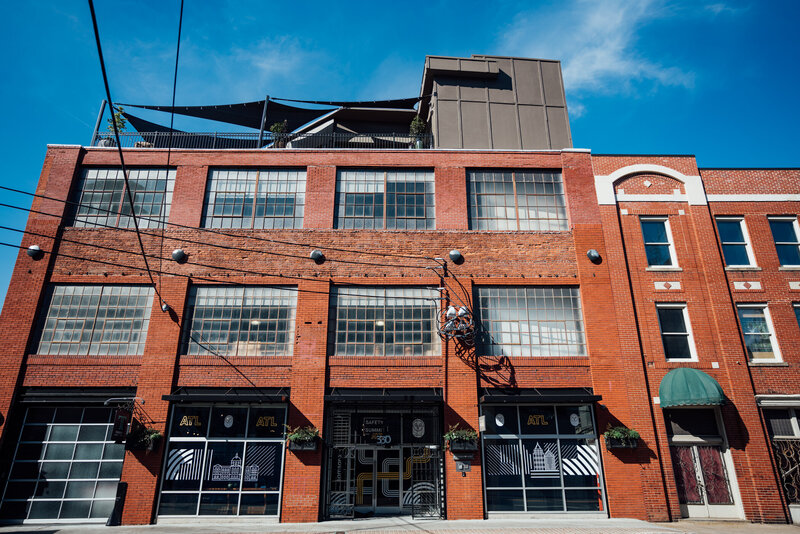This detailed photographic image captures an outdoor scene of a three-story, orangish-brown brick building. The photo is taken from a crouched position, looking upwards, which makes the building appear inclined. The facade consists of four large square windows in three rows on the left side, each window spanning nearly from floor to ceiling. Additionally, the lower level features two distinct sections separated by a doorway in the middle: on one side, there are what appear to be large glass windows, possibly indicating a commercial space, while the other side has smaller, regular windows.

The main entryway is characterized by double doors with white frames and windows at the center, highlighted by a green awning above them. Just above this doorway, an arch structure is noticeable, with a single window on both the second and third floors. Adjacent to the entrance, there's an entryway leading to what may be a lobby, marked by the unclear numbers 10 or 30 and the letter E, next to a sign with unreadable text.

High above, the roof features a grey structure resembling a shed, along with what appear to be grey-black tents. Shadows conceal some figures on the rooftop beneath the tarps, making their activities indistinct. The background showcases a beautiful blue sky with feathery clouds, adding a picturesque quality to the image. Window boxes adorn the columns outside the building, enhancing the architectural details. The specific angle and crisp outdoor setting of the photo emphasizes the building's imposing height and distinctive character.